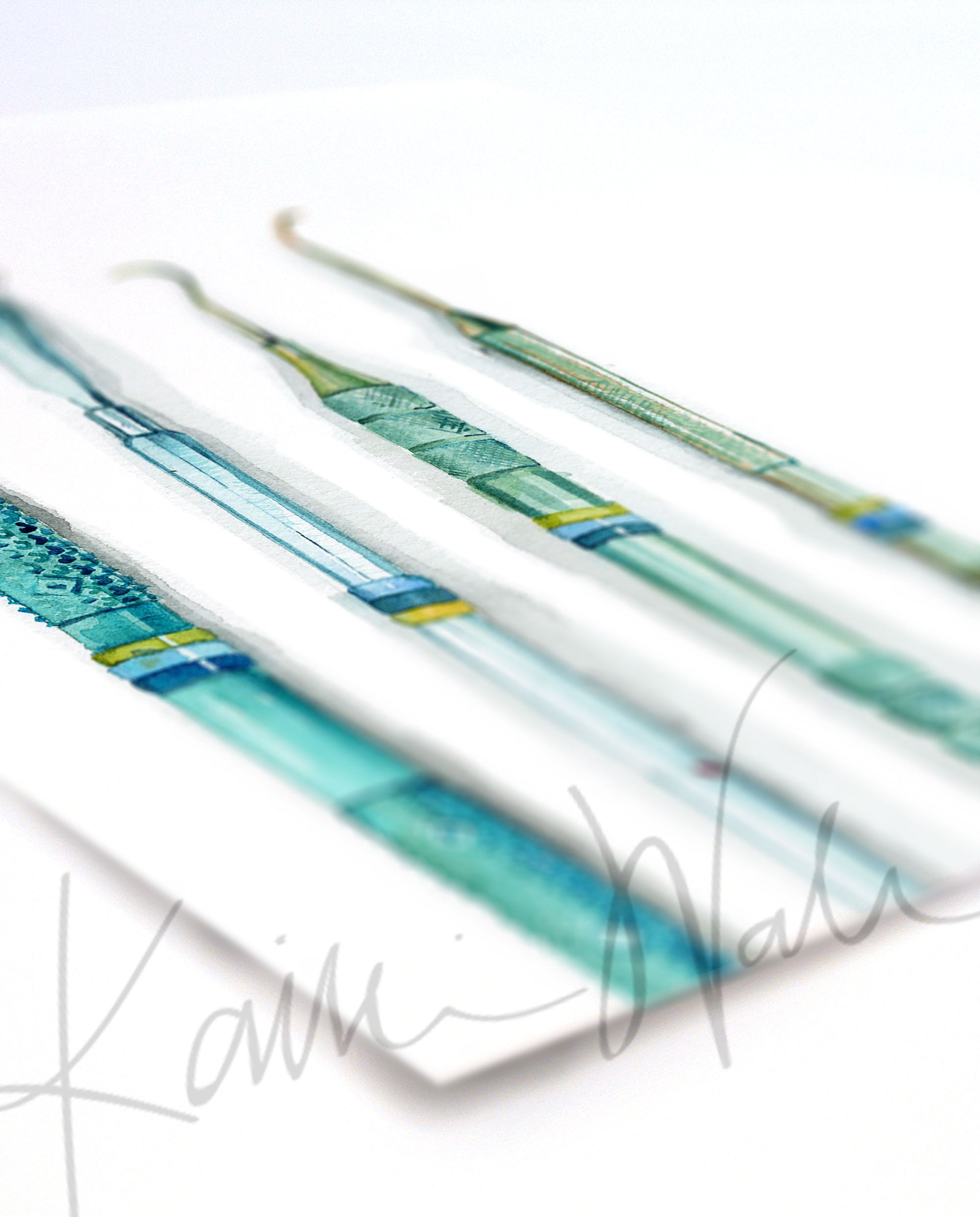This detailed close-up photograph captures a card laid flat on a white surface at an angle, revealing about 70% of the artwork. The image features four greenish-blue dental tools with yellow, light blue, and dark blue bands around their handles. The tools have textured grips and two of them, on the right, have hook-shaped scraping tips, the kind used in dental care. The leftmost tools are partially obscured, with their tops cut off. The colors of these tools include shades of blue, green, and possibly yellow, creating a mixed palette. A light gray, blurry watermark signature is visible across the lower portion of the image, with the name starting with a "K" and the last name starting with a "W", possibly reading "Kam Nala" or "Kyrie Watata". The card is placed on a blank white background, and a subtle shadow beneath the corner of the card differentiates it from the white surface beneath.